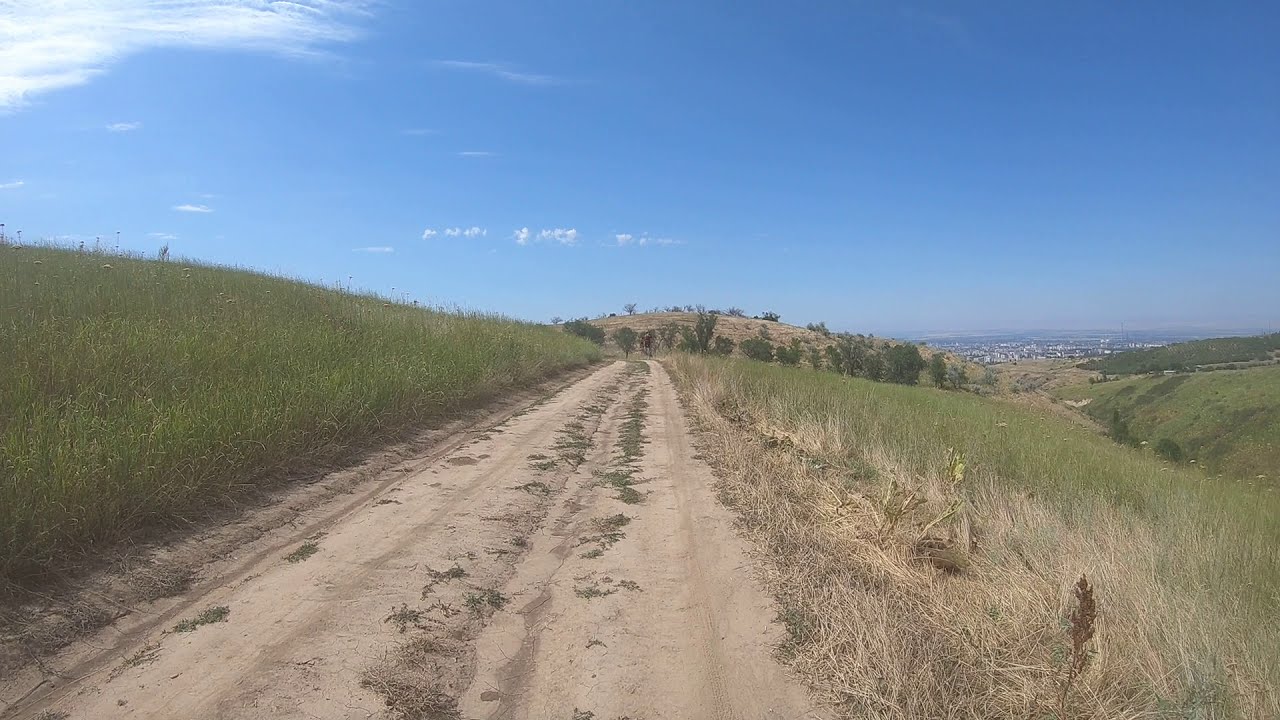The photograph captures a dirt road that stretches into the distance, perfectly centered and running vertically through the frame. The road, composed of brown or gray soil, has a notable dip down its center where rainwater often pools, creating a distinctive line. Flanking this line, remnants of dead grass or moss are visible. To the left, a verdant hill rises, densely covered in tall grass and weeds, while to the right, the land slopes downward into a valley also populated with weeds. The bright blue sky is peppered with wispy white clouds; on close inspection, faint skywriting can be discerned, though the letters are indecipherable. In the distance, multiple hills—some blanketed in trees—are visible, with one particular area giving way to a forest and farther still, a city skyline can be faintly seen. The overall scene exudes a sense of tranquil remoteness while hinting at civilization beyond the natural landscape.